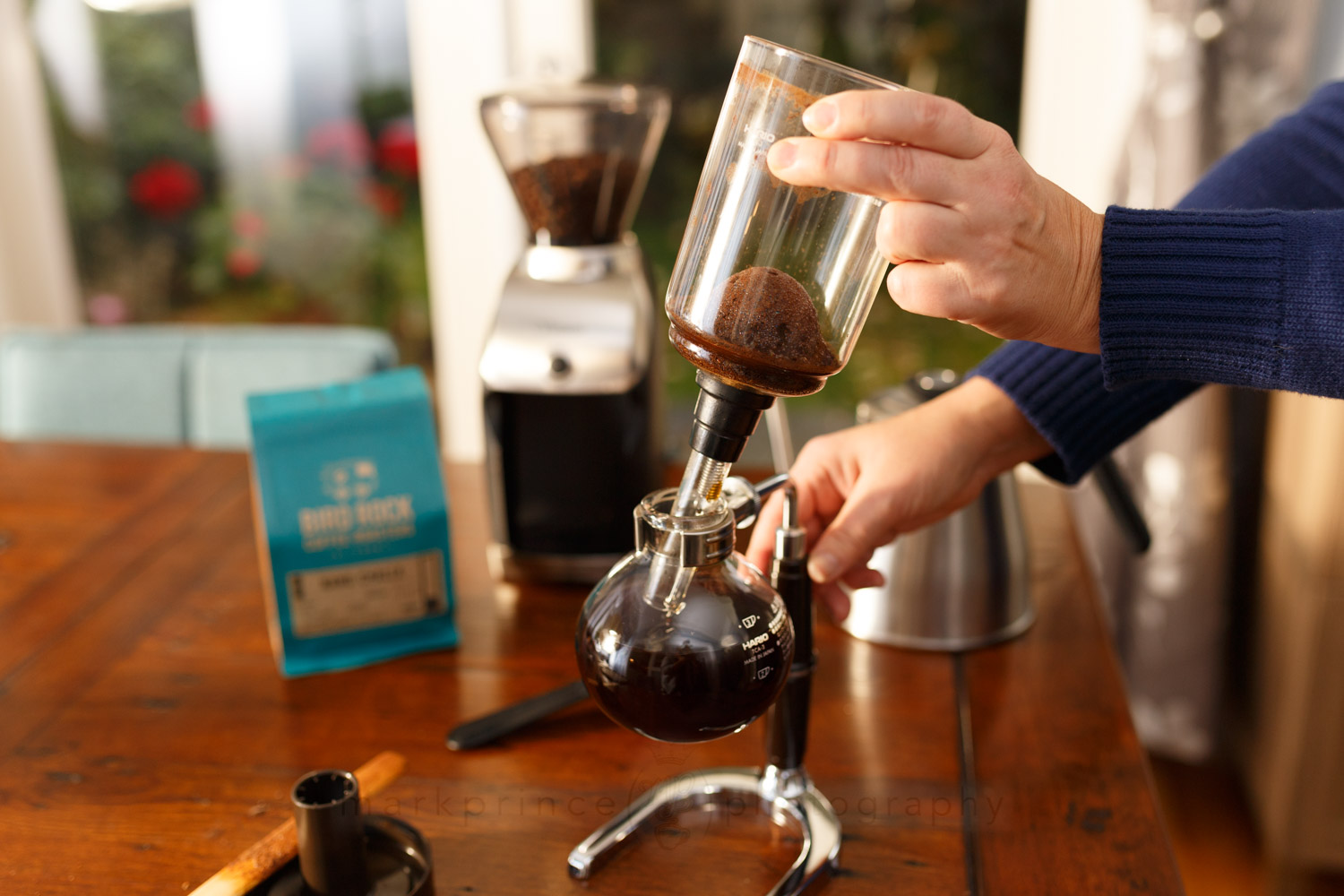In this photograph, a person is brewing coffee using an elaborate setup more commonly seen in a professional coffee bar than a typical kitchen. The visible portion of the person, from their forearms to their hands, is clad in a long-sleeved blue sweater. They are meticulously holding a cylindrical glass canister filled with damp ground coffee beans in one hand. This canister has a tube at its base, channeling into a small spherical coffee brewer. The brewer, resembling something out of a scientific laboratory, appears to be made of Pyrex glass and is affixed to a black and chrome horseshoe-shaped metal stand, which rests on a dark red wooden countertop. The meticulous arrangement also includes various coffee-making paraphernalia: a coffee grinder, a large metal coffee pot, a blue bag of coffee beans, and other unspecified items. Out the window in the background, flowers can be seen blooming, adding a touch of natural beauty to the scene.